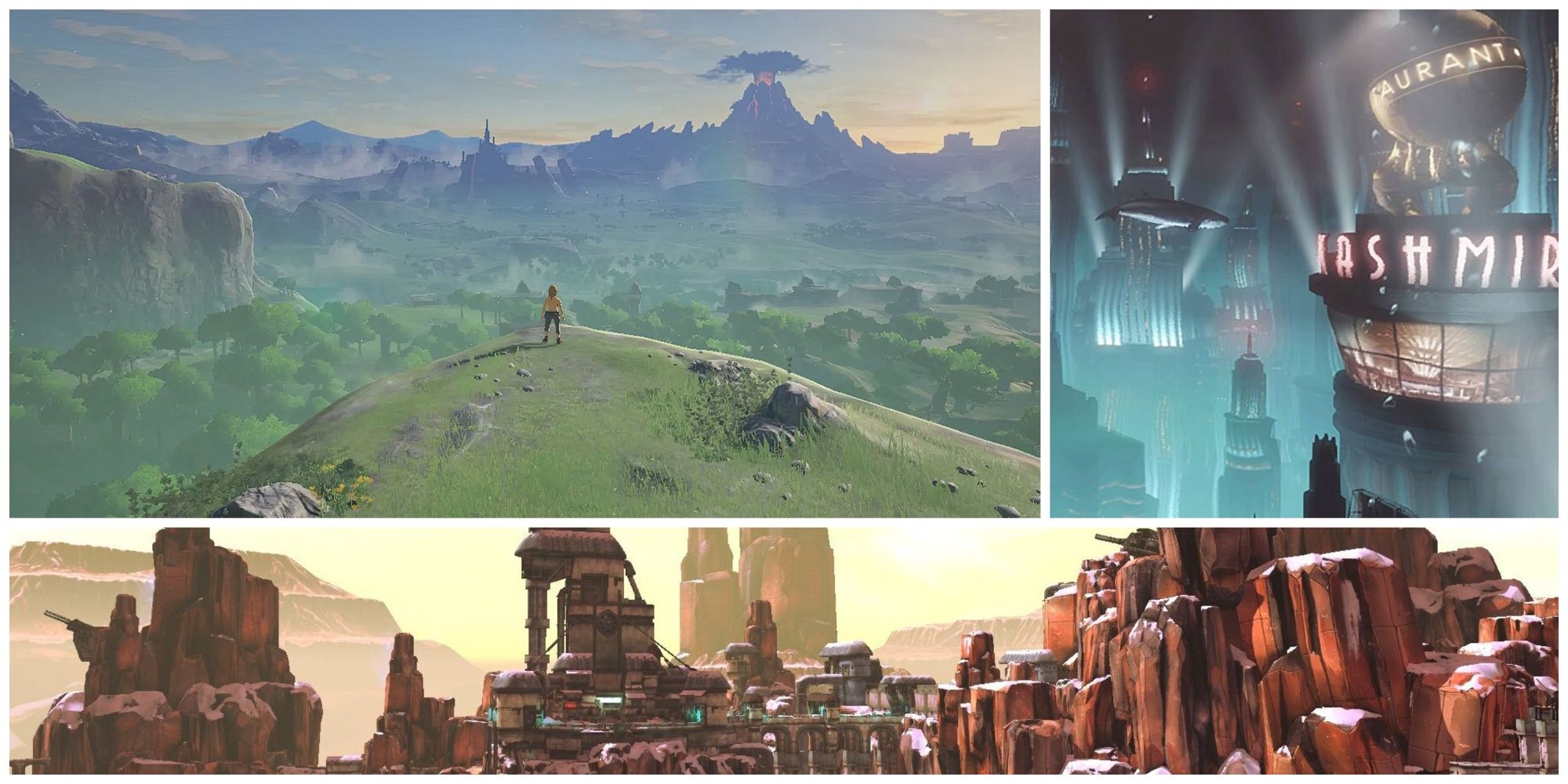The composite image features three distinct scenes from different video games, arranged in a two-by-one layout. 

- **Top Left:** A breathtaking, scenic valley framed by majestic mountains with lush forests and a distant, ominous volcano. This image strongly resembles the visual style and landscape from "The Legend of Zelda" series, specifically from the recent titles "Breath of the Wild" or "Tears of the Kingdom".

- **Top Right:** A futuristic, neon-lit scene showcasing a building adorned with the sign "Kashmir" and part of another sign hinting at a "restaurant". The environment is accentuated by spotlights and an extraordinary sight of a whale floating through the scene, suggesting a sci-fi or cyberpunk video game aesthetic.

- **Bottom:** A portrayal of a city's defense system laden with rocket launchers and various artillery, all enveloped in a distinct brown hue reminiscent of the Grand Canyon. This gives off a sense of a heavily fortified area within a barren, desert-like landscape.

Overall, the composite image appears to showcase a selection of vibrant and diverse video game worlds, possibly part of a promotional spotlight for different titles.